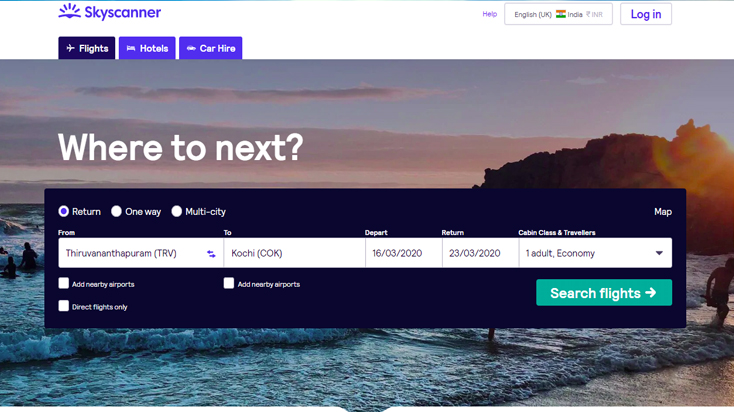The image displays a Skyscanner interface, a well-known travel booking platform. 

- In the top left corner, the Skyscanner logo is prominently displayed, with the company's name clearly visible. Directly below the logo, there are menu options for "Flights," "Hotels," and "Car Hire."
- On the top right, there's a hyperlink labeled "Help," and an option to select the language and region, showing "English (UK/India)" as the selected option. Next to it is the "Log In" button.
- Centrally displayed is a scenic photo of a beach, possibly captured around late afternoon or early evening, approximately at 6:30 p.m. Overlaid on the image is the prompt "Where to next?"
- Underneath this prompt, there are radio buttons for travel options, with "Return" selected. Other options include "One-way" and "Multi-city."
- The fields for travel details are populated as follows: departing from "Thiruvananthapuram (TRV)" and traveling to "Kochi (COK)." The departure date is set to 16.03.2020, with the return date on 23.03.2020.
- The travel configuration specifies "1 Adult, Economy Class," with a drop-down menu for adjusting these settings.
- Just beneath, there are additional options with checkboxes for "Add nearby airports," "Direct flights only," and "Add nearby airports" again.
- At the interface's bottom center lies a prominent green button labeled "Search flights," with a "Map" button immediately above it.

This detailed description encapsulates all interactive elements and visual cues present on the Skyscanner booking interface.